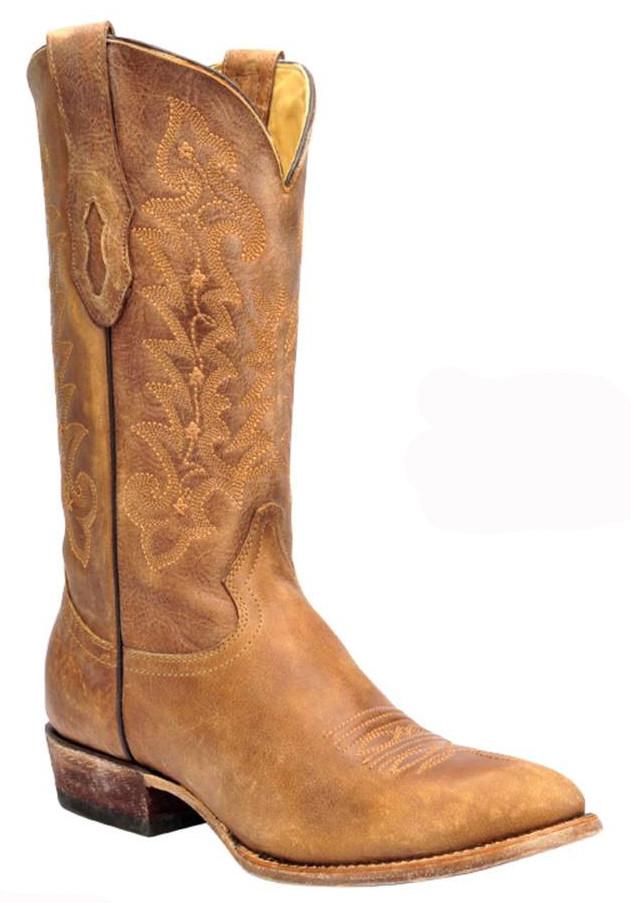This image features a single, well-worn cowboy boot photographed against a stark, pure white background, giving it a product display appearance. The boot is for the right foot and is made of light brown leather with slight wear markings, especially on the heel and toe areas. The boot has a distinctive medium to light brown color, transitioning to orange accents toward the toe. The sole is orangish brown and noticeably worn, with the interior lined in a yellowish material.

The boot is adorned with intricate detailing and patterns. A fine floral embroidery, featuring curved S-like patterns and leaf-like shapes, extends from the foot up to the top of the boot, which reaches just below the knee. This pattern includes what appears to be winding stems, small stars, and squiggly lines, adding depth and texture to the leather. The design is consistent on both sides of the boot.

At the top, the boot has a pair of functional straps, shaped almost like elongated triangles, which aid in adjusting and securing the boot. These straps are positioned above a thick black line that marks the boundary between the dark brown heel and the front of the boot. The boot's heel is slightly elevated, about half an inch, and is distinctively dark brown.

Overall, the boot combines classic cowboy aesthetics with delicate, detailed craftsmanship, making it both a functional and visually appealing piece of footwear.